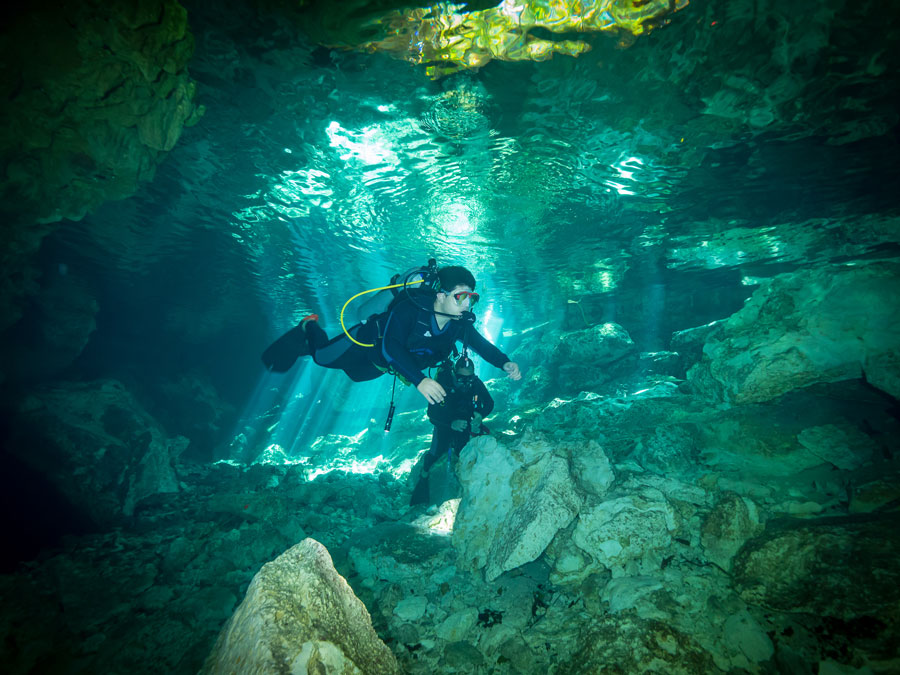In this underwater scene, two scuba divers are exploring what appears to be a submerged cave. Illuminated by a narrow beam of sunlight that trickles down from a small opening above, the divers navigate the shadowy, rocky environment. Overgrowths of vines and shrubs partially obscure the entrance, hinting at a small area where they might have entered the water. The dominant hues of the image are dark and murky, with no visible sea life, enhancing the sense of isolation and exploration. 

The scuba diver closest to the viewer, identifiable by his black hair, is swimming horizontally, donning a black wetsuit, black fins, and a dive tank with a yellow hose and a black mouthpiece. His companion, slightly in the background, stands upright on a rock, possibly adjusting his equipment or examining an object. The cavernous walls on either side of the frame reinforce the cave-like environment, adding to the adventurous and mysterious ambiance of the underwater expedition.